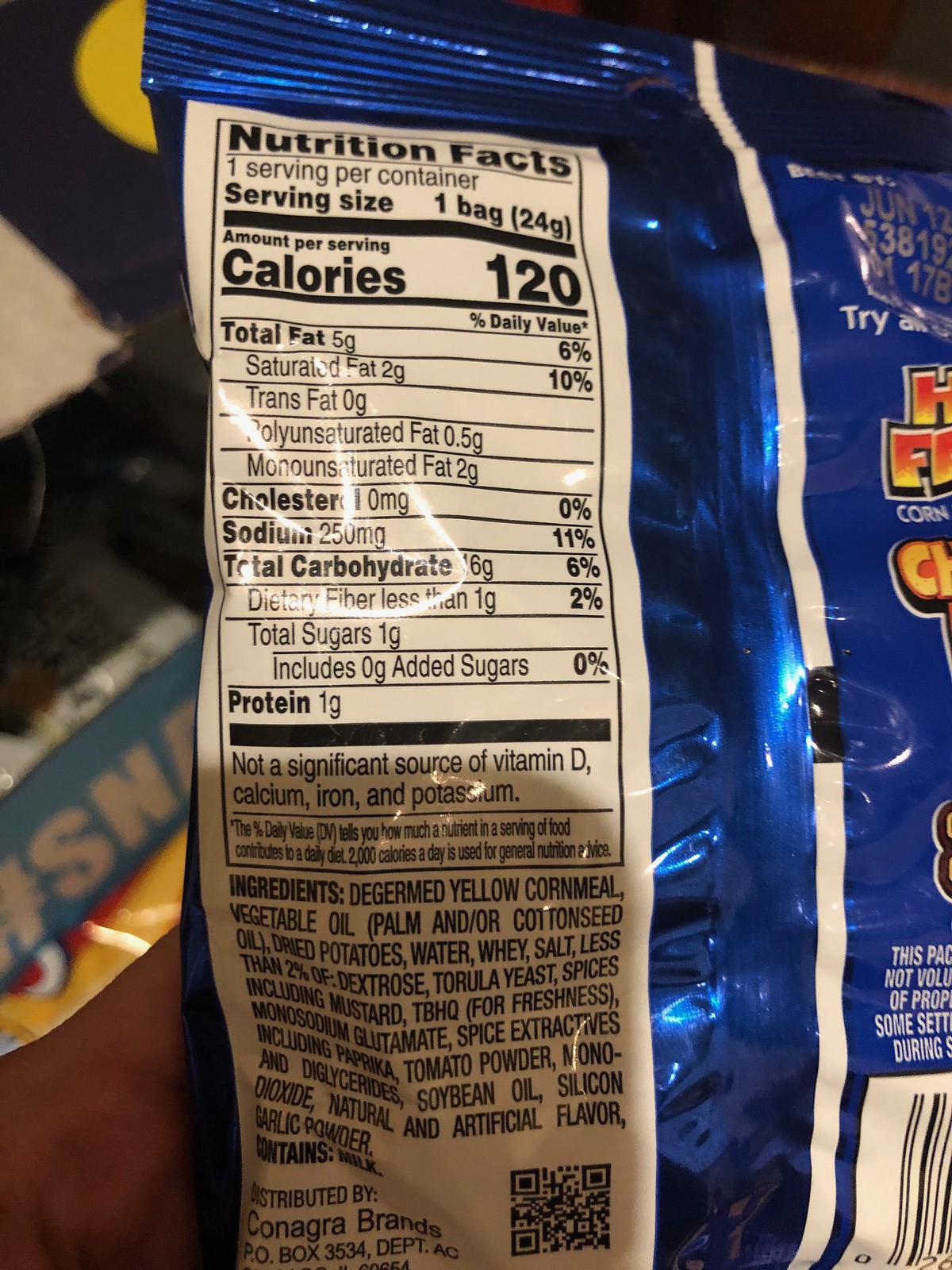In the center of the image is a snack bag set against a crispy, golden buttery background. The snack bag is sealed at the top, with nutrition facts prominently displayed on the lid. The bag contains one serving per container, each serving weighing 24 grams. 

The detailed nutrition facts per serving are as follows:
- Calories: 120
- Total Fat: 5 grams
  - Saturated Fat: 2 grams
  - Polyunsaturated Fat: 0.1 grams
  - Monounsaturated Fat: 2 grams
- Cholesterol: 0 grams
- Sodium: 23 grams
- Total Carbohydrates: 6 grams
  - Dietary Fiber: Less than 1 gram
  - Total Sugars: Less than 1 gram
- Protein: 1 gram

Ingredients for each serving include: corn oil, vegetable oil, palm oil, linseed oil, dried potatoes, water, wheat, salt, tortilla, beef, spices, clove mustard, peppercorns, peanut butter, mandarin oil, soybean oil, garlic powder, sugar, and other flavorings.

Additionally, there is a QR code on the right side of the bag, and an orange letter on the top right corner. The white letters spell out "core." The overall packaging design, coupled with the detailed labeling, communicates a well-thought-out snack product, ready to indulge your taste buds with its rich, buttery, and crispy flavor.